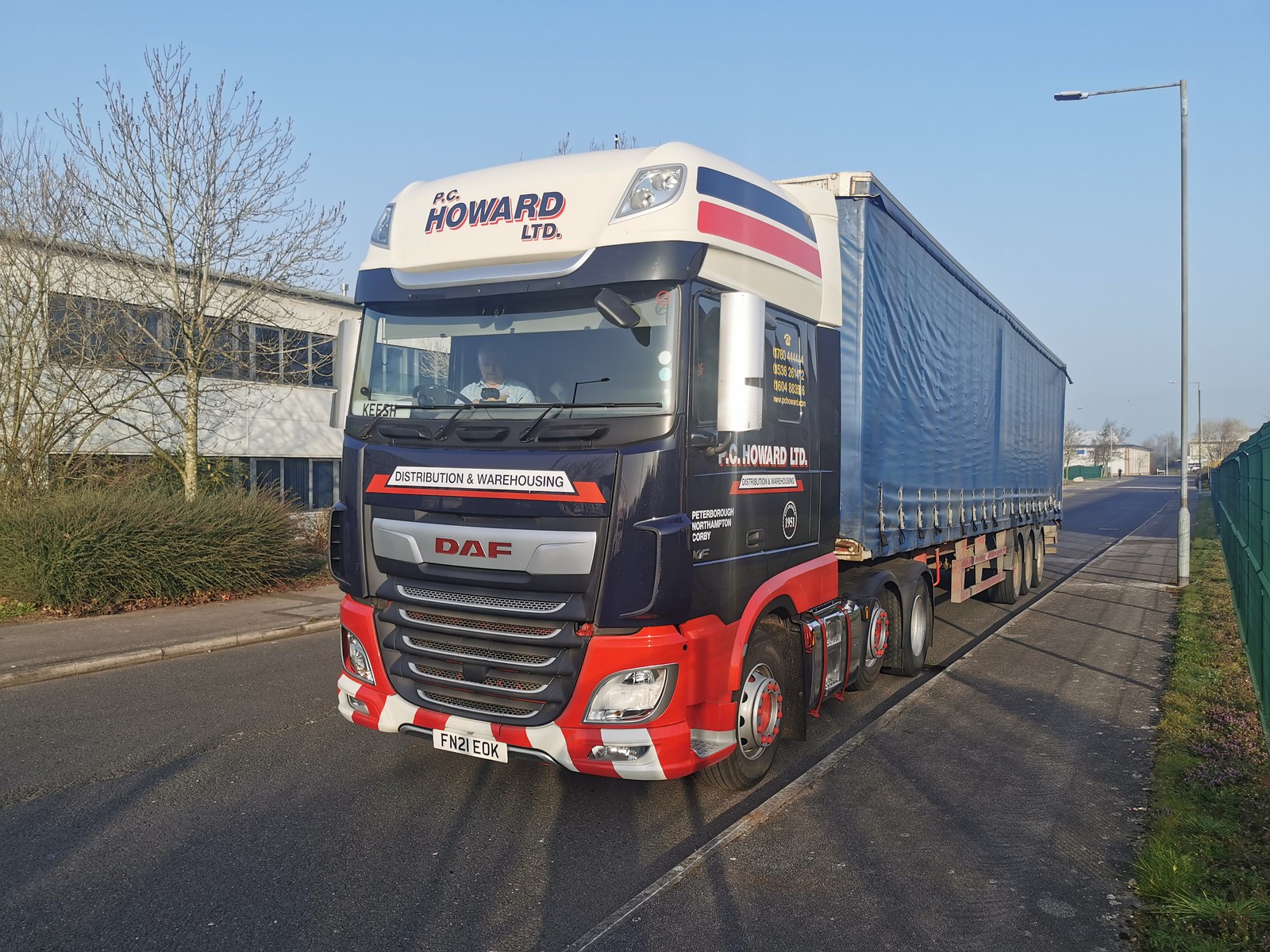This vivid image showcases a semi-truck belonging to PC Howard LTD on a bright, cloudless day. The truck is prominently displayed, facing towards us and angled to the left, driving on the left side of a street. The truck’s head features a striking combination of black and red, embellished with blue and red stripes along the sides, and white stripes accentuating the front bumper. The top of the truck’s cab prominently displays the name "PC Howard LTD" in blue letters. The trailer, covered in a blue or gray tarp, complements the color scheme.

The truck's cab also bears the logo "DAF" on its front grille, and there's further branding on the side door with "Howard LTD" in white letters. The license plate reads FN21EOK. The truck sits in stark contrast to its surroundings, which include a sidewalk, a couple of bare trees indicating it's winter, and a two-story building. There are also grassy columns and a light pole nearby, delineating the street’s edge.

A middle-aged male driver, dressed in a light-colored shirt adorned with some design, is seen inside the cab, focused intently on the dashboard or steering wheel. The street scene, the pristine blue sky, and explicit details on the truck and its surroundings underscore the sheer vibrancy captured in this image.